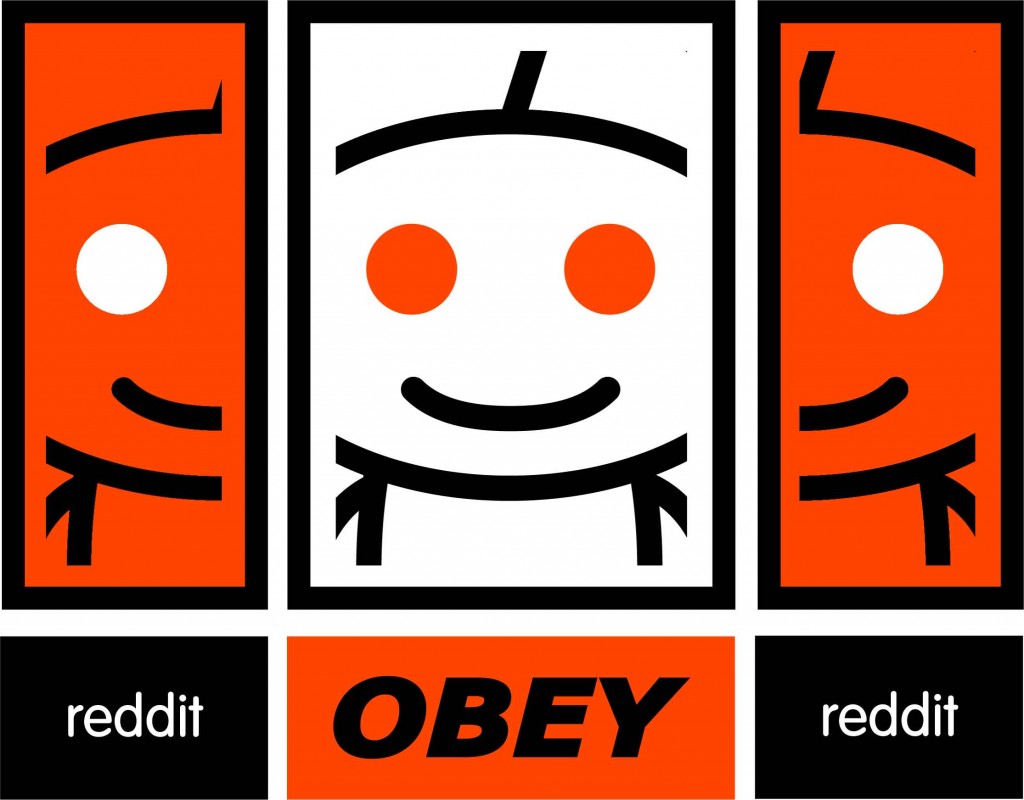In this image, created for the company Reddit, there are six distinct panels that come together to form a cohesive design. 

- **Top Left Panel**: This vertical block features a red-bordered square with a black padded border. Inside, the left-hand side of a simplistic face/body is depicted with a white dot for an eye and a small curved line for a smile.

- **Top Center Panel**: This section showcases a minimalist face on a white background with a black padded border. The face has two red dots for eyes and a smiling mouth, complementing the overall cheerful theme.

- **Top Right Panel**: Similar to the top left, this panel mirrors the face design with a white dot for an eye and a smiling mouth. The face is circular with a small body beneath it.

- **Bottom Left Panel**: A black block with the word "reddit" written in white text.

- **Bottom Center Panel**: Here, bold black text spells out "obey" on a red background, prominently positioned in the panel.

- **Bottom Right Panel**: Mirroring the bottom left panel, this block also features the word "reddit" in white text on a black background.

Collectively, the image is designed to represent Reddit, showcasing three simplistic faces of potential contributors or users at the top, followed by the brand's name "reddit" and the bold statement "obey reddit" at the bottom. The design emphasizes the brand's identity through its distinctive visual elements.